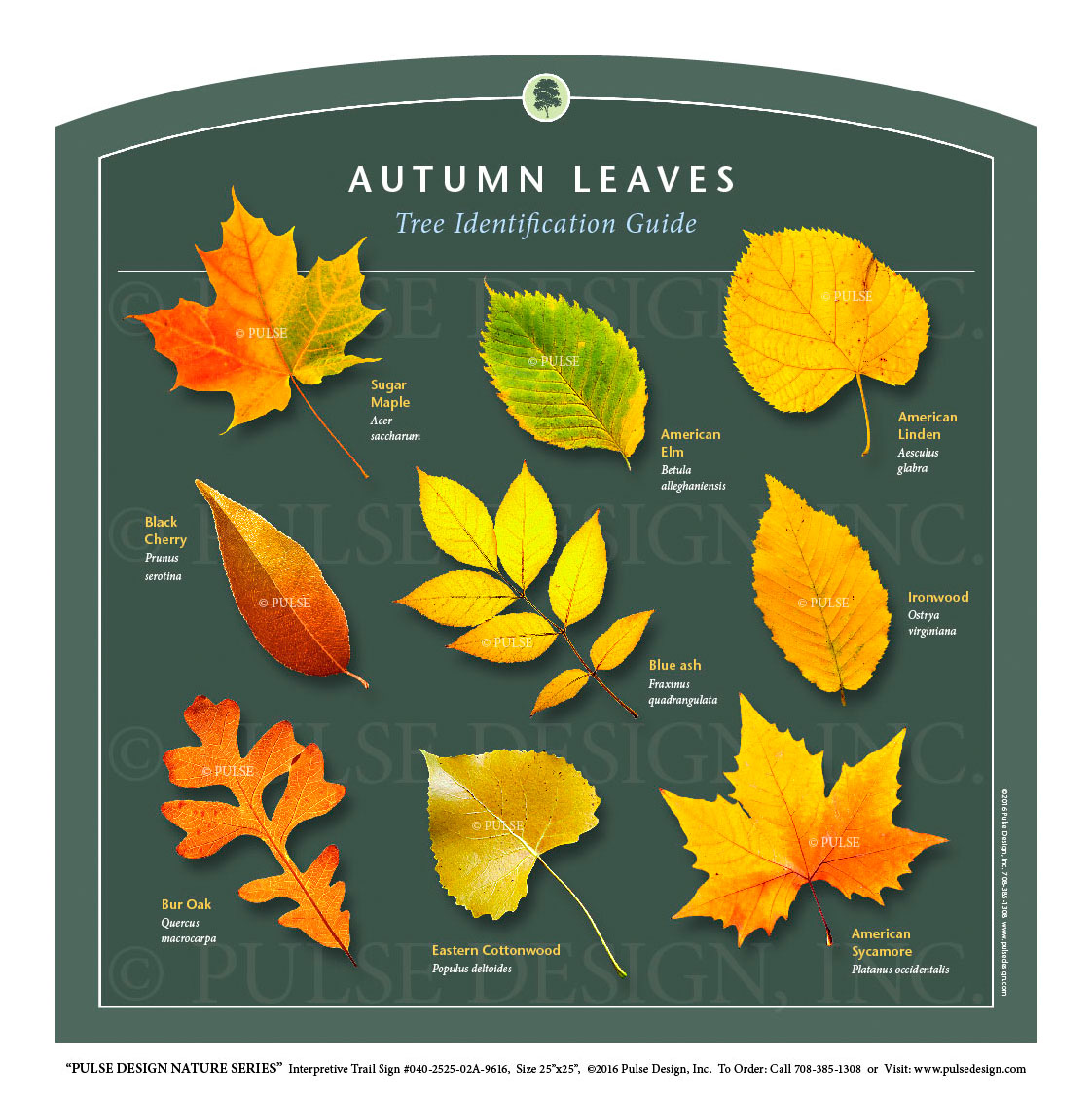The illustration is a detailed design poster titled "Autumn Leaves Tree Identification Guide." It features nine different types of autumn leaves: Sugar Maple, American Elm, American Linden, Black Cherry, Blue Ash, Ironwood, Burr Oak, Eastern Cottonwood, and American Sycamore. Each leaf is depicted with its distinctive outline and shape, showcasing a vibrant palette of reds, yellows, oranges, and occasional greens, set against a dark hunter green background that enhances the vivid colors. The leaves’ common names, such as the Sugar Maple and American Elm, are highlighted in yellow lettering, while their Latin names are presented in white. This carefully crafted guide combines educational content with artistic design, making it suitable for use as a textbook illustration or a nature-themed poster, and is part of a series called "Post Design Nature Series."